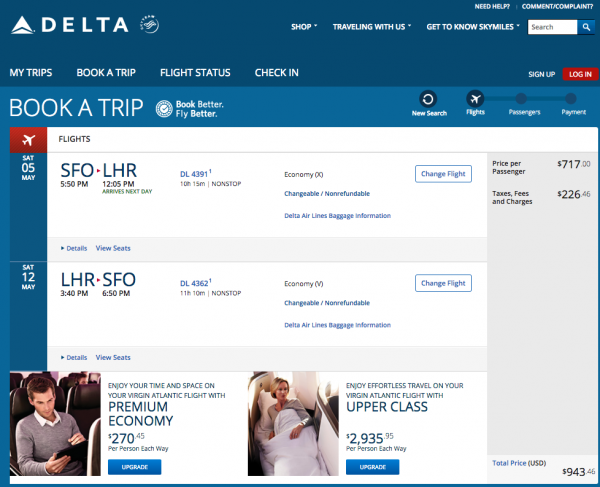**Descriptive Caption for Screenshot of Flight Booking Website**

The image is a screenshot of a flight booking website featuring a dark blue header at the top. On the left side of this header, there is a logo composed of two nested triangles: one steeper white triangle and one shallower white triangle, separated by a thin blue line. To the right of the logo, the word "DELTA" is displayed in white, all-caps text. Further to the right, there is an indistinct white circular logo, which is too blurry to identify clearly.

Following some empty space, the header features white all-caps navigation links: "SHOP," "TRAVELING WITH US," "GET TO KNOW SKY MILES," and a search bar with a white magnifying glass icon inside a blue square at the far right. Gray placeholder text within the search bar reads "SEARCH." Above these links, two lines of smaller white text read "NEED HELP?" and "COMMENT / COMPLAINT?" separated by a thin white line.

At the bottom of this header, left-aligned links in smaller white all-caps text include "MY TRIPS," "BOOK A TRIP," "FLIGHT STATUS," and "CHECK IN." On the right-hand side, there is a "SIGN UP" link accompanied by a red rectangular button with rounded corners that reads "LOGIN" in white text.

Below the header, the body of the page has a lighter blue background. In the top left corner, large, thin white text reads "BOOK A TRIP." Adjacent to this text is a blurry circular white icon. To its right, two lines of text state "BOOK BETTER, FLY BETTER," where "BOOK" and both instances of "BETTER" are bolded, but "FLY" is not. This section is followed by some space and various icons, with an arrangement indicating available flight options below.